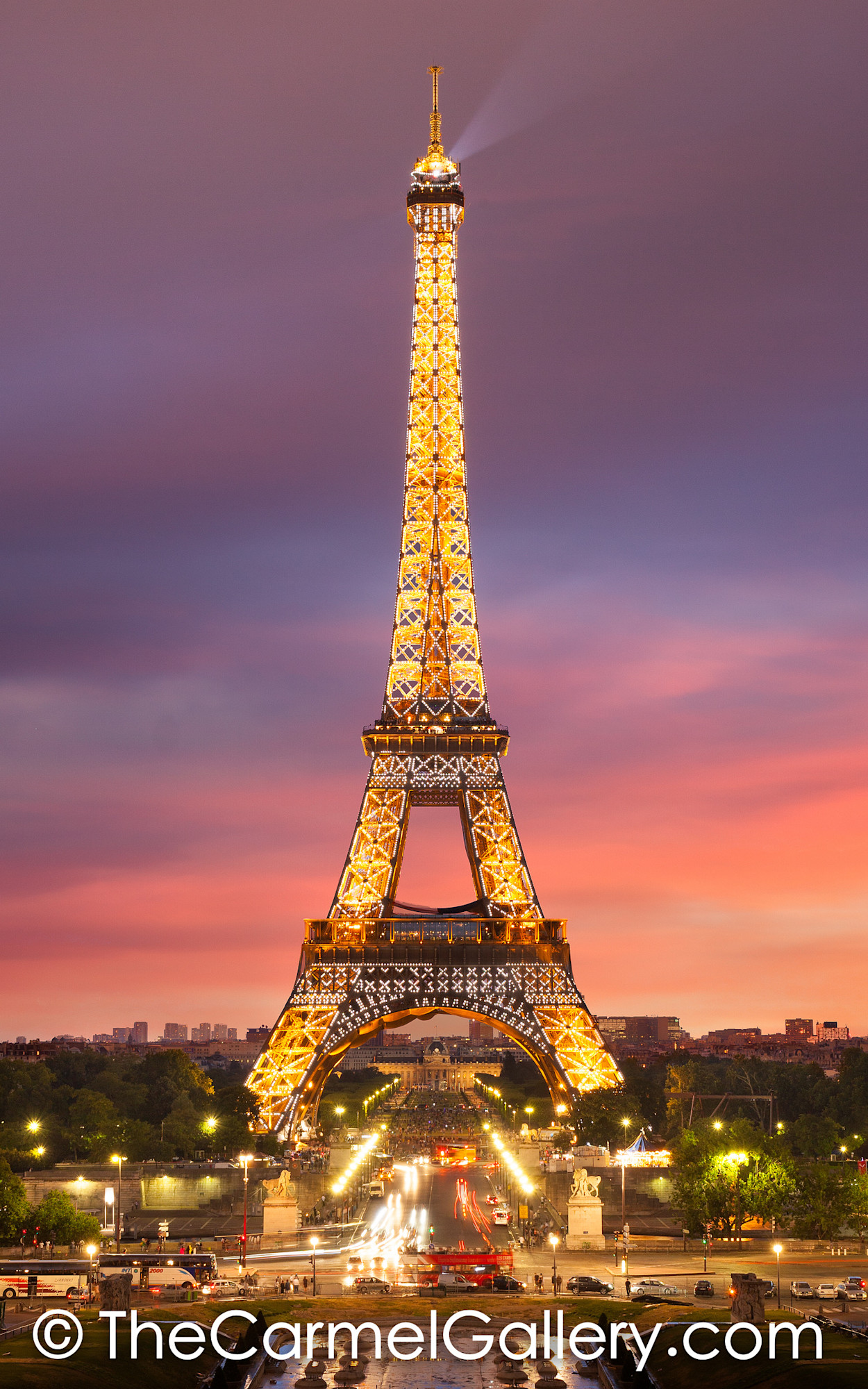The photograph showcases the iconic Eiffel Tower in Paris, beautifully illuminated with golden lights from its base to its pinnacle. Set against a stunning twilight sky, the hues transition from the warm oranges and pinks of a just-set sun at the horizon to deeper blues and purples higher up. The bustling avenue beneath the tower is also brightly lit, with streetlights lining the road and a few vehicles including tour buses and a distinctive red double-decker bus visible. Surrounding the base are a mix of Parisian buildings—shops, houses, and possibly some skyscrapers—which appear darker in contrast to the glowing tower. On either side of the avenue, which passes directly under the Eiffel Tower, you can spot some green trees and a couple of stone statues. A faint copyright in white text, "thecarmelgallery.com," is visible at the bottom of the image. The overall scene is vibrant yet serene, a perfect blend of natural and artificial illumination capturing the essence of Paris at twilight.